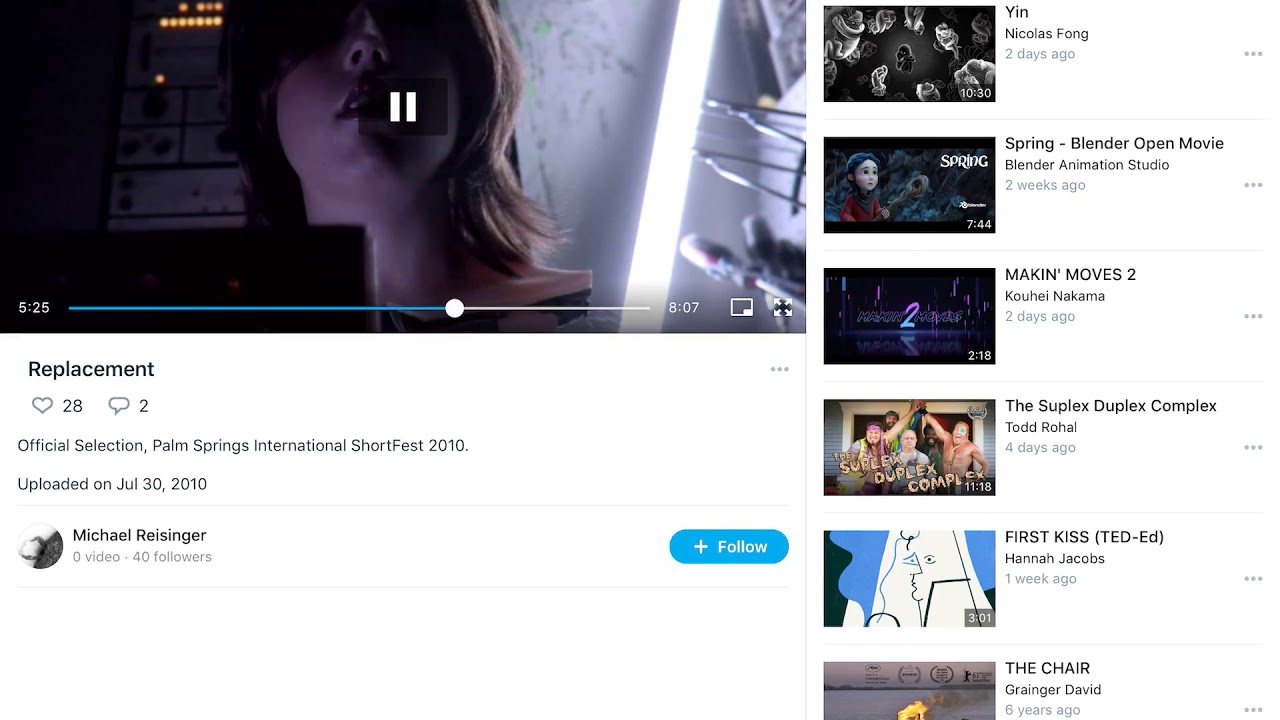This detailed screenshot from a video titled "Replacement" captures a key frame at 5 minutes and 25 seconds into the playback. In the image, a woman with shoulder-length, wavy auburn hair and side bangs tilted to the left gazes slightly upward, her collarbones prominently visible. Her nose appears slightly upturned. The background features a warm, orange glow, possibly from lit-up stereo equipment.

The video player interface is clearly visible, with a timeline marking the progress of the video. The elapsed time is highlighted in light blue, contrasting with the unviewed portion of the timeline, which remains white. Below the video, the title "Replacement" is prominently displayed, accompanied by interactive icons: a black-outlined heart indicating that 28 people have liked the video, and a speech bubble showing there are 2 comments.

The description reads, "Official Selection, Palm Springs International Short Fest 2010. Uploaded on July 30, 2010." Beneath this, a user icon displaying a partial eyebrow and eye signifies the video's uploader, Michael Reisinger. Next to his name, a light blue oval icon with a white plus symbol and the word "Follow" invites viewers to subscribe to his content.

To the right, a sidebar lists additional videos, partially visible: "Yin," "Spring Blender Open Movie," "Making Moves 2," "The Suplex Duplex Complex," "First Kiss," and "The Chair," though the last thumbnail is cut off midway.